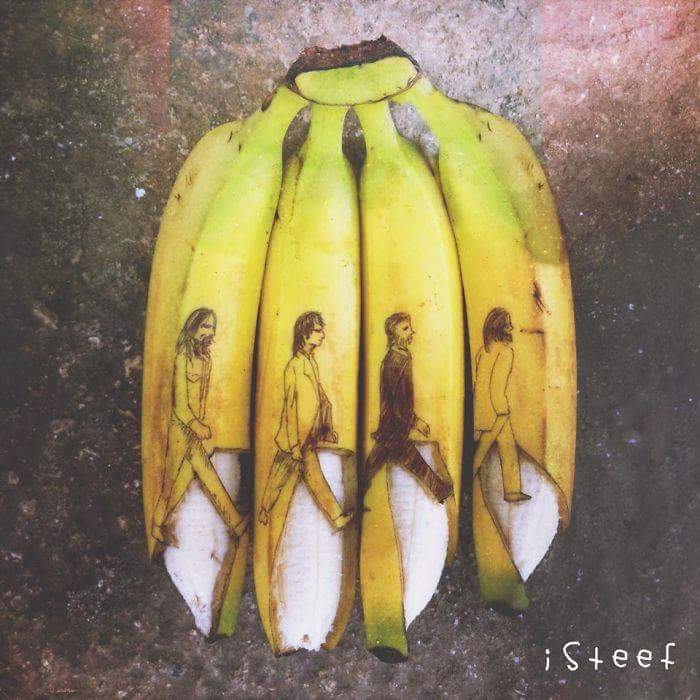The image showcases an artistic rendition inspired by the Beatles' iconic "Abbey Road" album cover, creatively depicted using four bananas. Each banana features a finely detailed, hand-drawn figure of a Beatle member, expertly positioned to mimic the famous crosswalk scene. The bananas are slightly peeled at the bottom, revealing their white interior, which cleverly represents the crosswalk stripes. The bananas, mostly yellow with hints of green and minor bruising, are still attached at their stems, arranged centrally against a textured, dark gray surface. The background appears cement-like with areas of lighter gray near the top and subtle pinkish hues around the edges. In the bottom right corner, the watermark "iSteef" is inscribed in white text, featuring a lowercase 'i' followed by an uppercase 'S' and the other letters in lowercase.